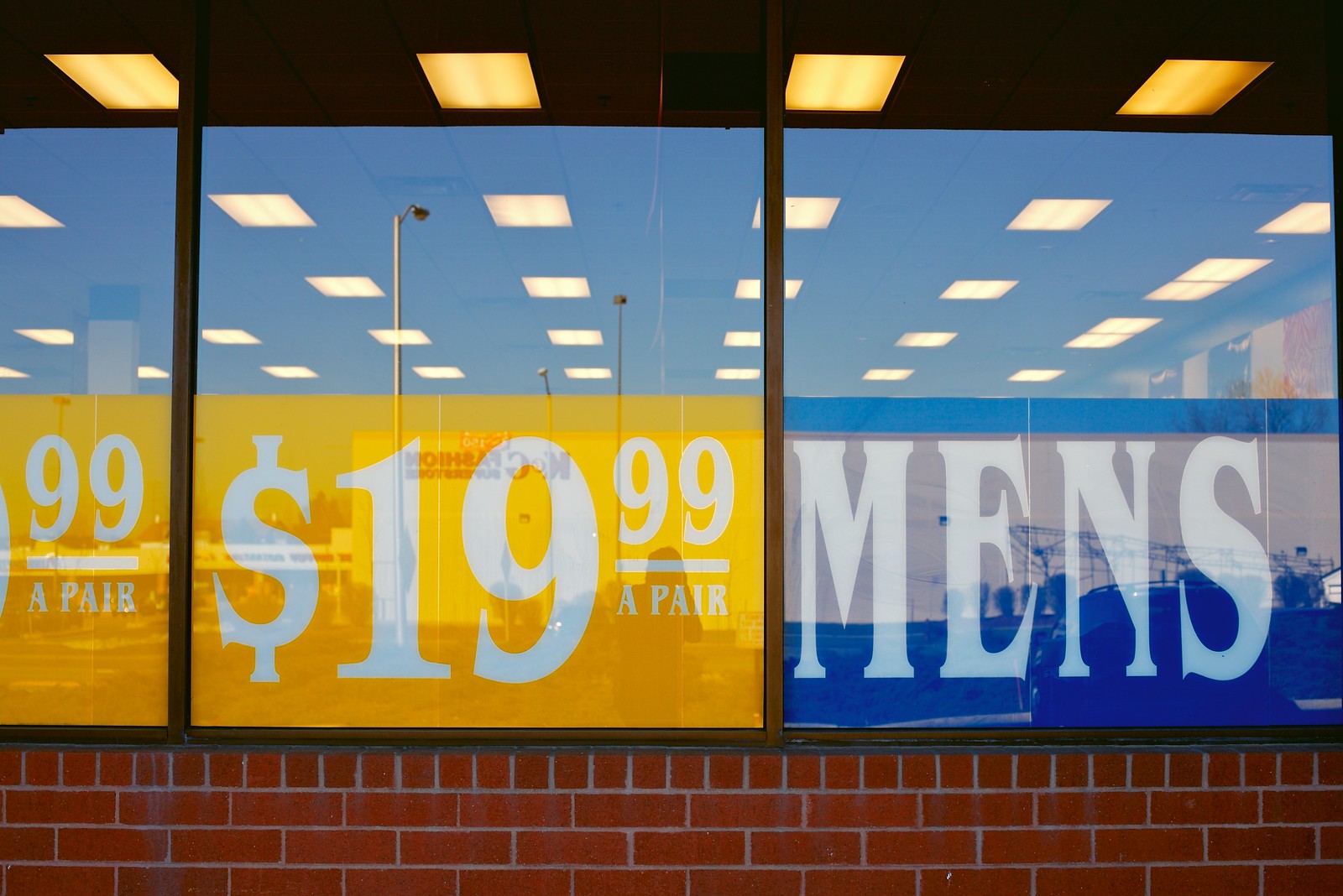The image features an expansive display of glass panes. The interior background showcases a tiled ceiling adorned with light fixtures, creating a well-illuminated space. Several pillars add to the structural elements visible within the frame. To the far right, colorful banners can be seen, along with the reflection of the photographer. The front of the image prominently features glass with two noticeable price squares: one yellow square on the left with "99 a pair" and a blue square to the right indicating "$19.99 a pair." Further right, the word "Men's" appears. The scene reflected in the glass includes a detailed landscape with a finger crane on the right, various cars, an industrial setting featuring poles and signposts, buildings in the distance, and a brick base bordered with white cement.